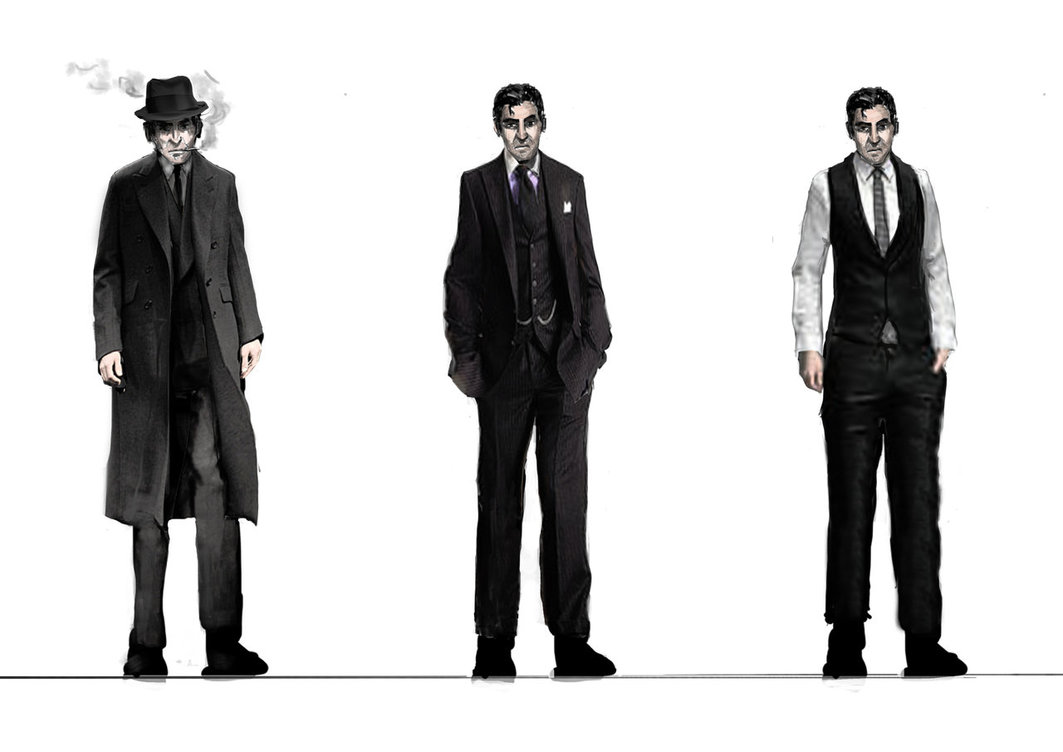The image is a detailed color illustration in landscape orientation showcasing a man in three distinct stages of clothing, all facing the viewer in a comic-style yet detailed rendition. Each depiction of the man emphasizes different attire, but all share the same serious expression.

On the far left, the man, who appears Caucasian, is wearing a knee-length black duster jacket and a black top hat, resembling a fedora. He is smoking a cigarette, with smoke curling around his face, and is dressed in gray pants and a suit jacket.

In the center, the same man is illustrated with his hands in his pockets, donning a black suit jacket layered over a black vest, a white dress shirt, and a black tie. He has curly black hair and maintains the same serious expression.

On the right, the man is dressed more casually, without the suit jacket, in a white long-sleeve dress shirt, a gray tie, a black vest, black pants, and black shoes. The illustration is primarily black and white with spot color, adding to the visual interest and detailed presentation of the man's attire.